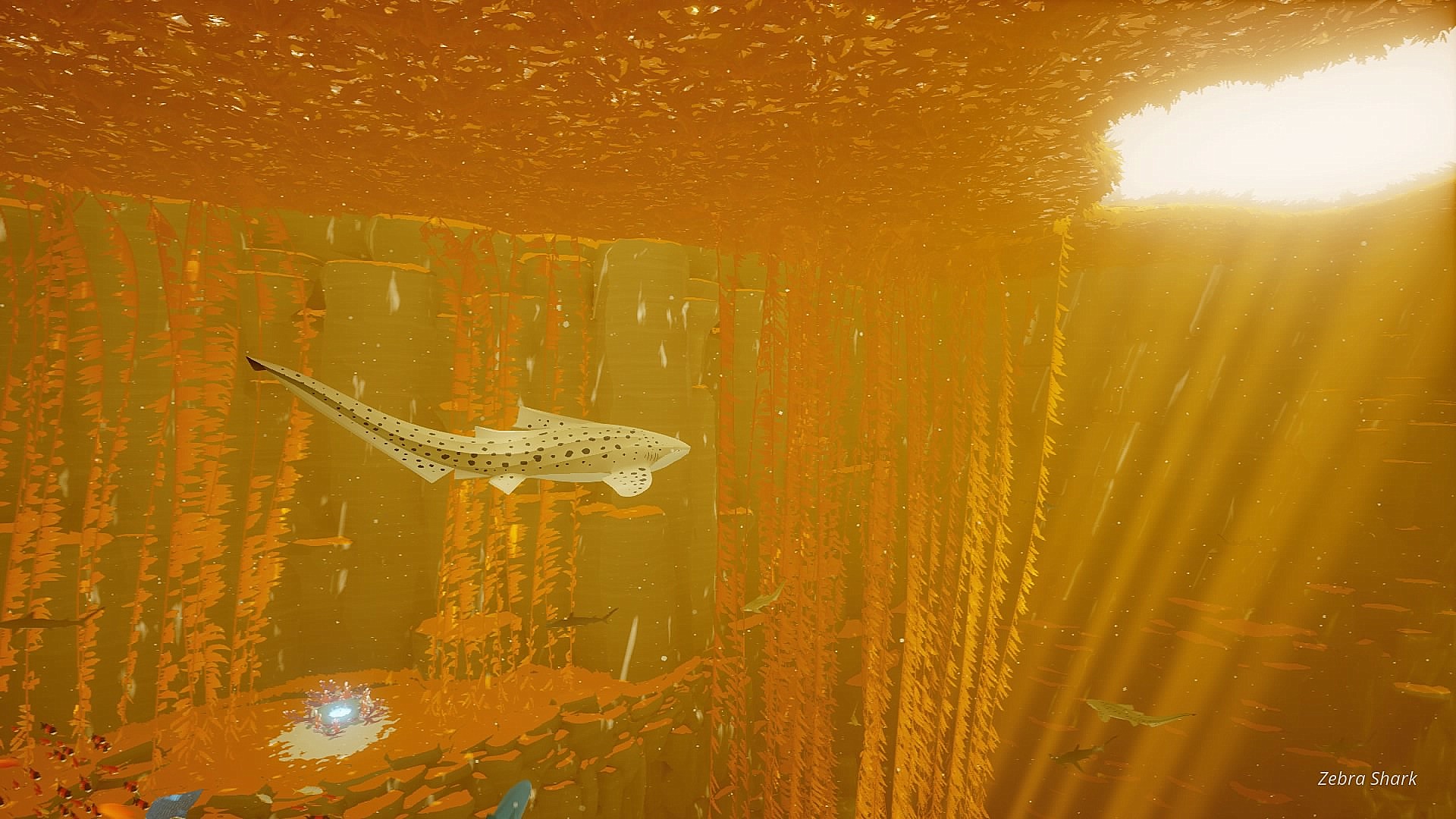Here is a refined and detailed caption based on the provided description:

---

A vividly colored, slightly blurry or overexposed underwater scene, possibly an illustration or an infrared photograph, showcases a small zebra shark. The image is predominantly orange, with hints of green possibly representing seaweed or underwater vegetation. The shark, located just off-center towards the left, stands out with its white body adorned with black spots. The bright, unusual coloration suggests infrared imaging, setting a unique and striking backdrop for this marine subject.